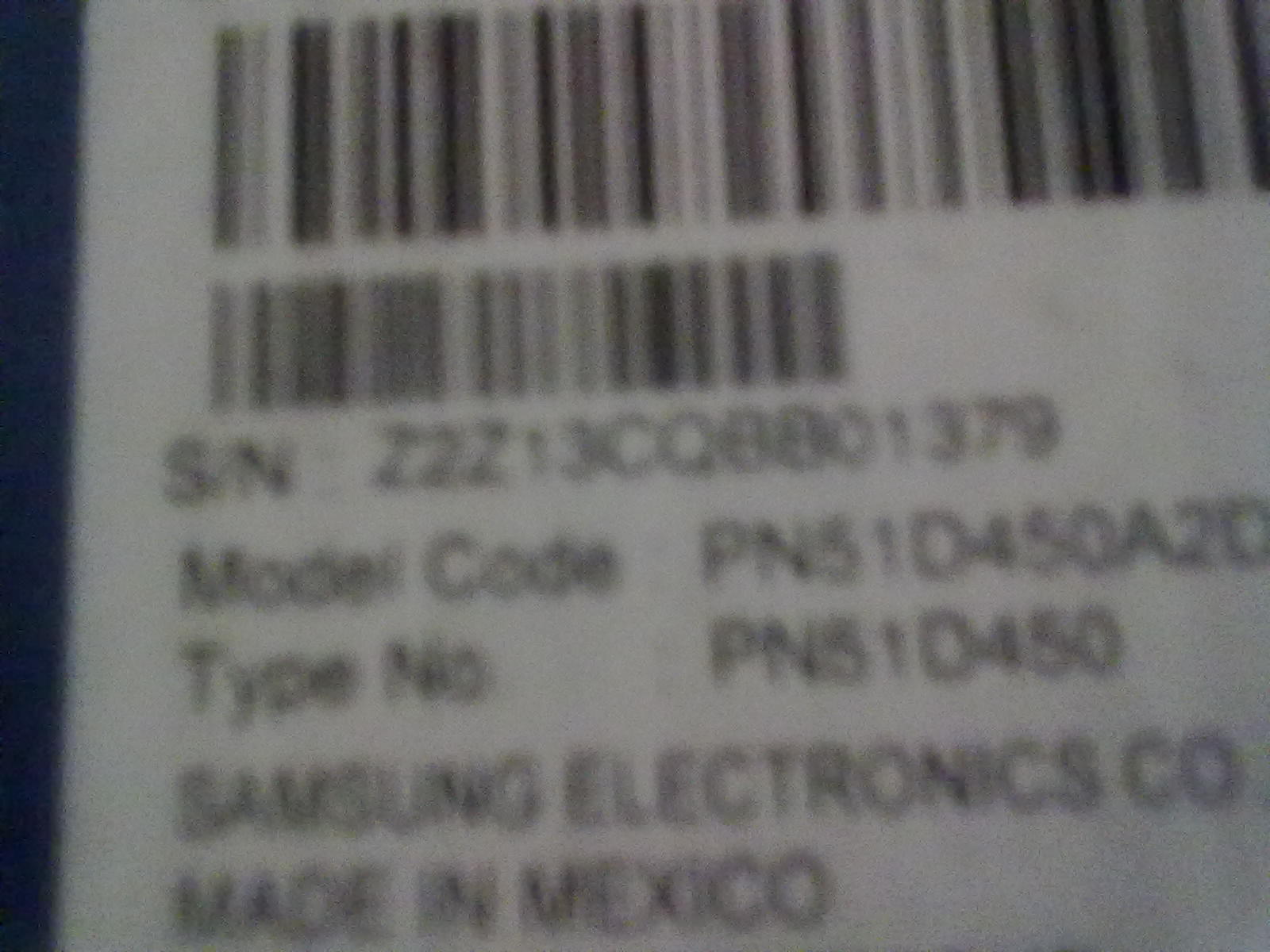A somewhat blurred, black-and-white photograph captures the back of a product, showcasing a series of identification details. At the top of the image, there is a barcode, followed immediately by a serial number, a model code, and a type number. Despite the blurriness, the text is still legible, providing crucial information such as the manufacturer's name, "Samsung Electronics Company," and the product's origin, "Made in Mexico." The focus is slightly off, and the image is tilted slightly to the right, but all key details are discernible amidst the blur.